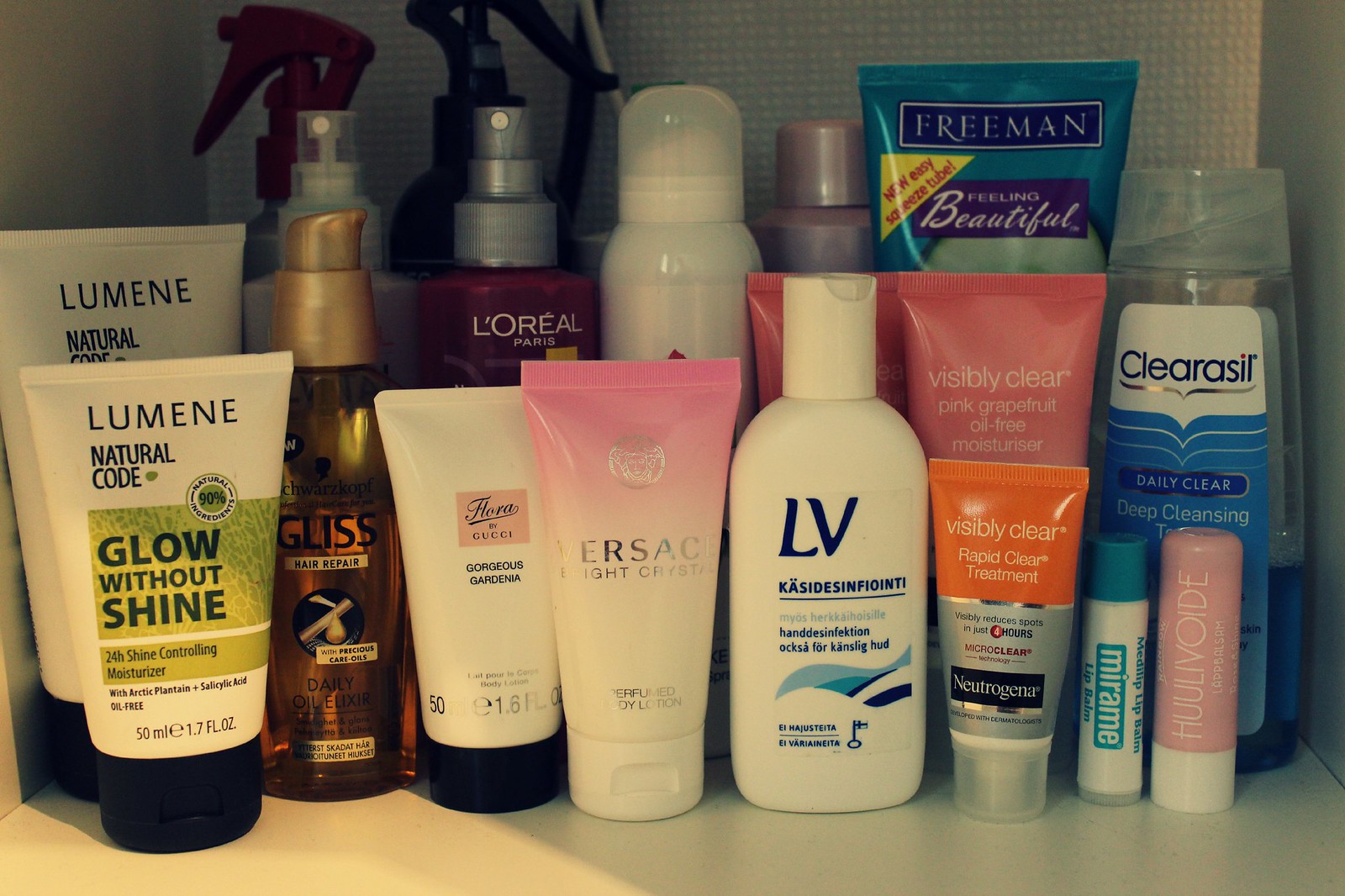The photograph captures a meticulously organized collection of beauty products arranged on a white shelf inside a cabinet. The cabinet itself is mostly white, with sidewalls cast in a slightly darker gray shadow, and a back panel adorned with a textured, small grid-like pattern of raised square bumps. This visually appealing backdrop sets an orderly stage for the products.

In the back left corner, two tall spray bottles stand prominently with two power cords extending down from their bases. Positioned in front of these are an array of taller bottles, mostly equipped with misting spray tops. This middle row features a diverse palette of colors, predominantly white, complemented by splashes of red, gray, and blue.

The front row showcases shorter bottles, many designed as squeeze bottles with thin plastic squeeze tubes on top capped with flat bottom lids. Among these, two small chapstick-type tubes stand upright in the lower right corner, adding to the assortment.

The variety of products includes several aimed at acne treatment, along with hair repair, conditioner, and moisturizer items. Visible brand names among this curated selection include L'Oreal, Lumene, Clearasil, Freeman, Mirame, and LV, reflecting a range of skincare and haircare solutions.